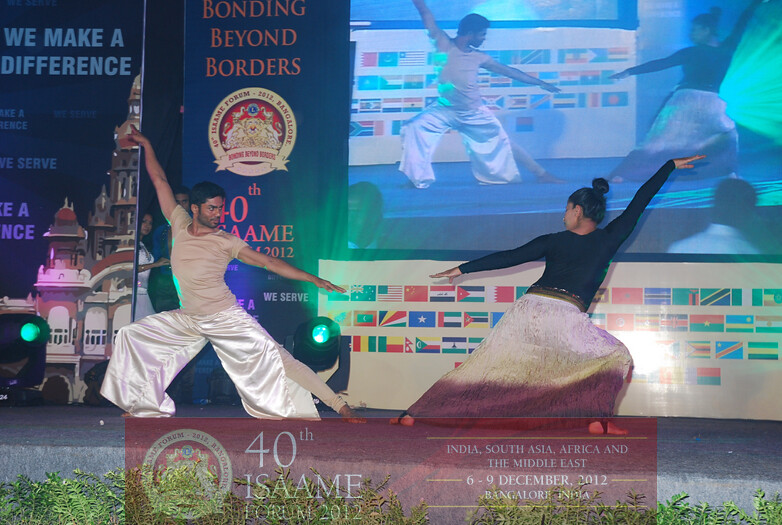In this vibrant outdoor photograph, a man and a woman, both appearing to be Indian, are striking a dynamic, dance-like pose on a stone or cement stage. The man, positioned on the left, has short black hair and a bit of a beard. He is dressed in a tan t-shirt and white palazzo pants with splits on the sides, revealing a beige leotard that extends down to his ankles. He extends his right arm up and behind him while his left arm reaches down and to the right. His left leg is outstretched, mirroring the fluidity of his movement.

On the right, the woman stands with her back towards the camera and her head turned left, looking at the man. She has her hair tied up in a bun and wears a long black sleeved shirt paired with a flowing white skirt that features a purple edge. Her left arm extends outward to the left, and her right arm is raised and pointing back. Their arms and legs create an expressive narrative between them, evoking a sense of intricate choreography, perhaps indicative of a sophisticated dance routine or martial art form.

In the background, a large screen replicates their current pose, reinforcing the synchronicity of their performance. Above them, a banner reads "Bonding Beyond Borders," adorned with various national flags on a white background, symbolizing a cultural or international event. Below the stage, a red sign with white letters declares "40th ISAAME Forum 2012" and details the event's location and dates: "India, South Asia, Africa, and the Middle East, 6 to 9 December 2012, Bangalore, India." The entire scene is alive with rich colors and intricate details, highlighting the cultural significance and elegance of their presentation.